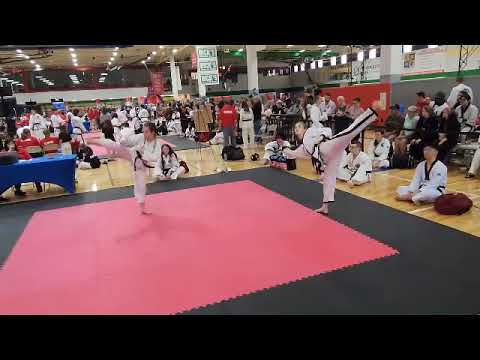In a bustling indoor gym, a captivating karate tournament unfolds. The focal point of the image showcases two young girls performing intricate jujitsu poses on a distinctive red mat surrounded by a larger black mat. Both girls, donned in traditional white karate uniforms with black belts, exhibit impressive high kicks: the girl on the left kicks forward with her right leg, while the girl on the right kicks back with her left leg. They both face towards the camera, their movements synchronized yet not directed at each other, suggesting a demonstration rather than a sparring match.

Encircling the performers, four children sit cross-legged on the ground, also dressed in white karate gis, embodying the disciplined spectatorship common in martial arts events. Behind them, a sea of onlookers watches intently from both sides and the back of the gym, delineated from the performance area by black poles. The audience includes many individuals in similar karate attire, reinforcing the event's competitive atmosphere. A man in a red shirt with white lettering, possibly a referee or organizer, stands out among the crowd, adding to the official nature of the event.

On the left side of the image, a blue table is visible, possibly serving as a judging or registration station. The backdrop is filled with a flurry of activity and multiple signs, hinting at the large scale and organized nature of this karate gathering.